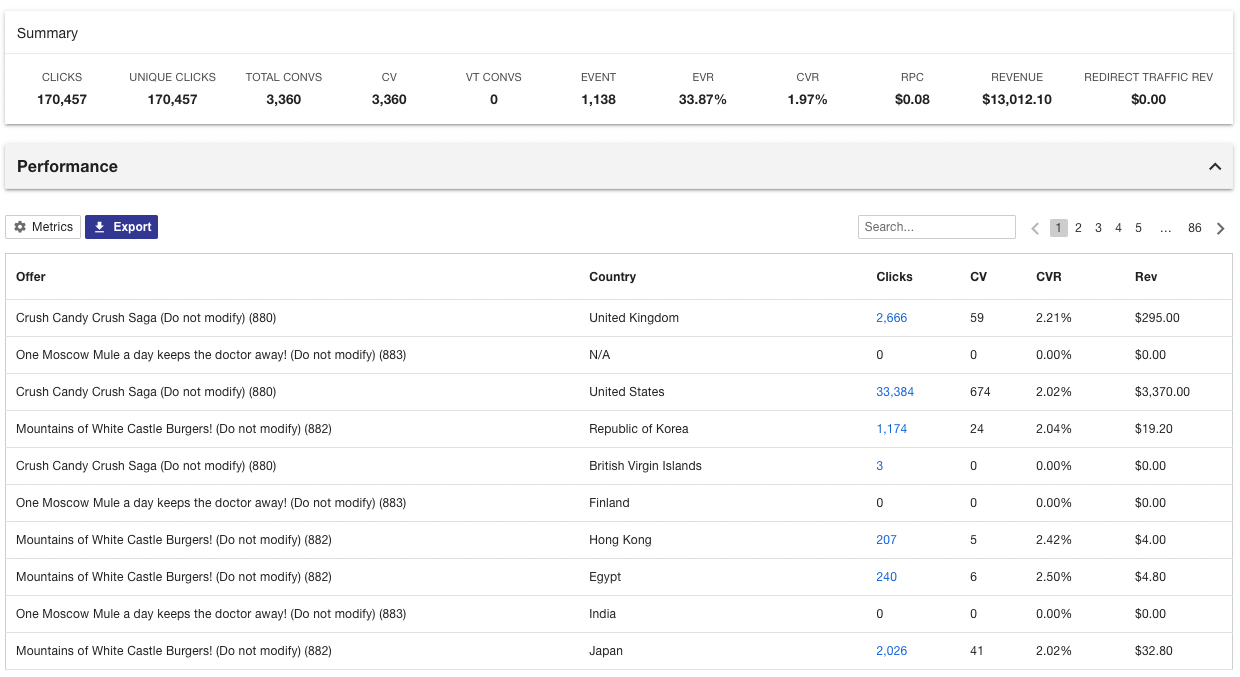The image is a screenshot of a data analysis dashboard. In the upper left section, the heading "Summary" is followed by a series of data metrics including clicks, unique clicks, total, comms, CV, VT comms, event, EVR, CVR, RPC, revenue, and redirect traffic revenue. Below this, there is a "Performance" section. On the left side beneath "Performance" are two buttons labeled "Metrics" and "Export." To their right is a search bar, accompanied by pagination tabs numbered one, two, three, four, five, and then ellipsis, ending at 85. 

Further down, there is a chart with columns labeled "Other Country", "Clicks", "CV", "CVR", and "REV". The left side of the chart features a list of entries, the first being "Candy Crush Saga." Following this are repetitive entries in the sequence: "One Moscow Mule a Day Keeps the Doctor Away", "Crush Candy Crush Saga", "Mountains of White Castle Burgers", and this sequence repeats several times. The final entries listed are again "One Moscow Mule a Day Keeps the Doctor Away" and "Mountains of White Castle Burgers."